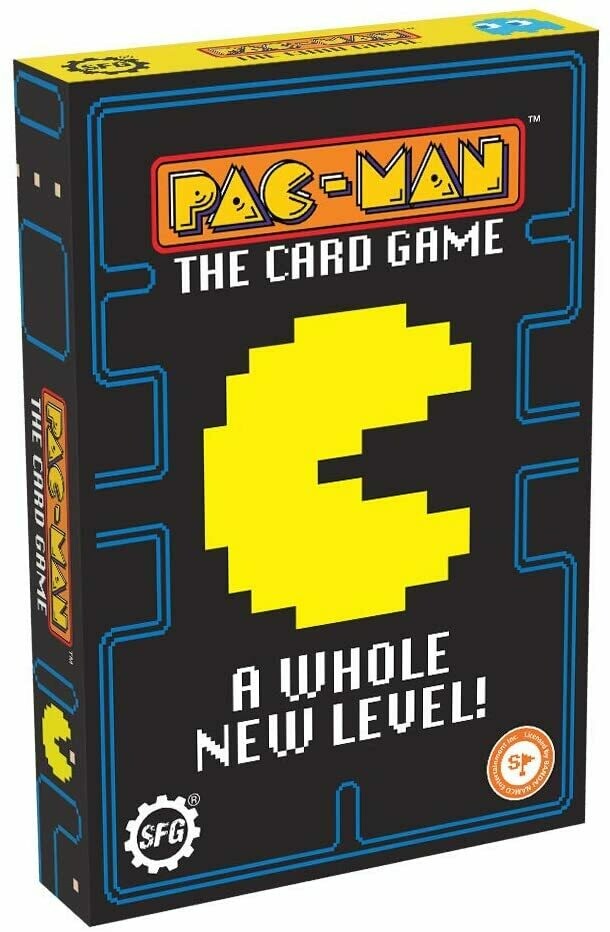The photo depicts a dark blue cardboard game box standing on end, titled "Pac-Man: The Card Game." The design on the front mimics the iconic Pac-Man maze, outlined in neon blue. At the center is a digitized yellow Pac-Man with its mouth open, facing right. Below the Pac-Man image, the phrase "A Whole New Level" is prominently displayed in a block style reminiscent of classic Pac-Man text. The top of the box is yellow, and along the side, the title "Pac-Man: The Card Game" is repeated. In the lower-left corner, there's a white stamp with the initials "SFG" inside a gear-like circle. Meanwhile, on the right side of the box, a partially visible circular symbol contains the letter "S."